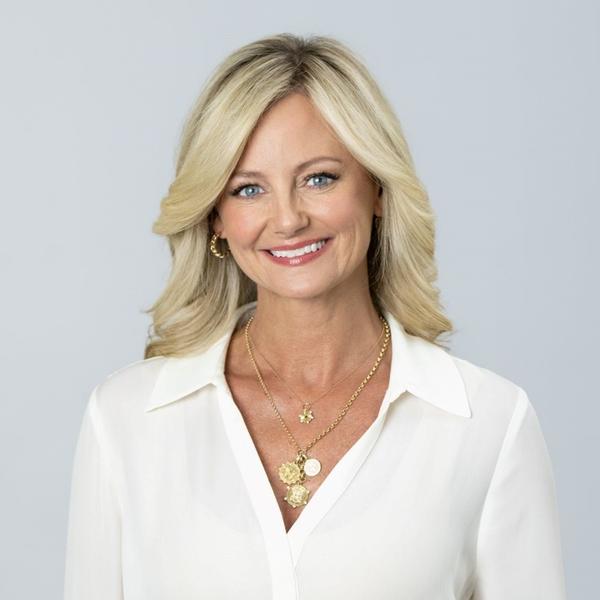The photograph features a middle-aged blonde woman with shoulder-length hair and striking blue eyes, smiling warmly at the camera. She is adorned with two necklaces: one shorter chain with a star-shaped pendant, and a longer chain with three circular discs. Complementing her look are hoop earrings and understated red lipstick. She is dressed in a white blouse, standing in front of a blue background, giving the impression of a professional headshot or portrait. Her confident and familiar expression adds a touch of elegant maturity to her appearance.